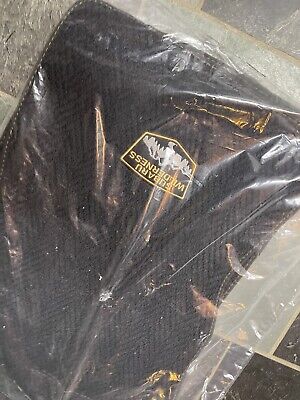The image showcases a black mesh item, possibly a piece of clothing or a car interior part, encased in a slightly torn and wrinkled plastic bag. This bag is placed on a slate gray and black tiled floor, which may be marble or concrete with distinctive golden grout. The light illuminating the scene comes from the top right, casting reflective highlights on the plastic. The black item within the bag features precise hand stitching along the edges and bears a five-cornered patch intricately embroidered in yellow, with "Subaru Wilderness" written on it. Below the text, the patch also depicts white mountains with a small trail running toward them, adding a rugged outdoor theme to the item.